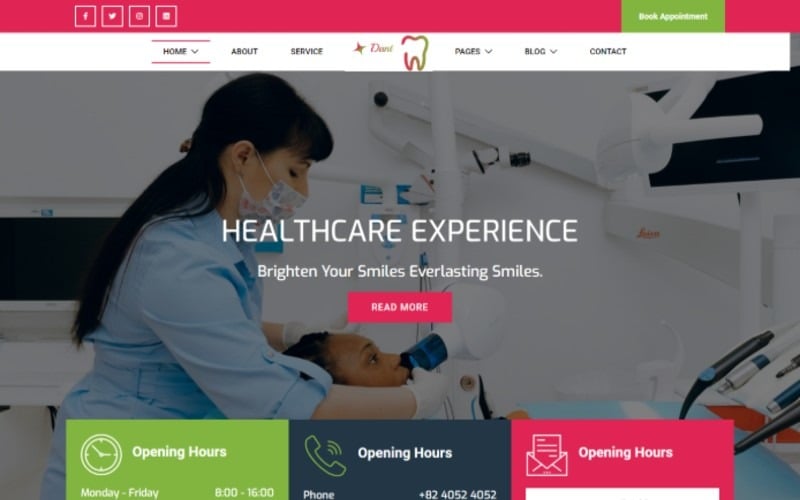A screenshot captures a healthcare website with a predominantly purple theme. The top bar is purple, featuring green text that reads: "Book Appointments," alongside links for "Home," "About," "Services," "Places," and "Contact." A section called "Healthcare Experience" aims to "brighten your smiles" and "everlasting smiles," highlighted further by a pink rectangular button with white text that says "Read More."

In the main visual section, a dentist is seen attending to a young girl in a dental chair. At the bottom of the website, the opening hours are displayed three times in different color schemes: green, dark blue, and pink, although the layout appears inconsistent.

The upper left corner of the screenshot contains small, hard-to-read icons for Facebook, Twitter, and what looks like an email icon. Notably absent is a clear company logo or name to identify the healthcare provider.